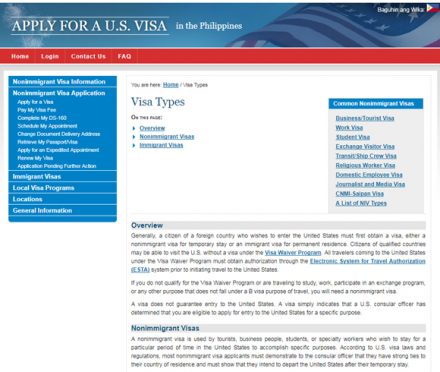This is a detailed screenshot of a U.S. visa application or information page. At the top of the page, a blue banner prominently features an American flag waving in the background. The banner contains large white text that reads "Apply for a U.S. Visa," with a decorative line above and below the text. Just to the right of this text, it specifies the location: "in the Philippines."

Below the banner is a red navigation bar with four buttons, though the first button is difficult to read. The second button is labeled "Log In," followed by "Contact Us" and "FAQ." A blue sidebar runs along the left side of the page and contains various white links for further navigation.

The main content area of the page has a white background and is centered around information about "Visa Types." To the right of this section, there appears to be a list of additional links, enhancing the page's navigation and accessibility.